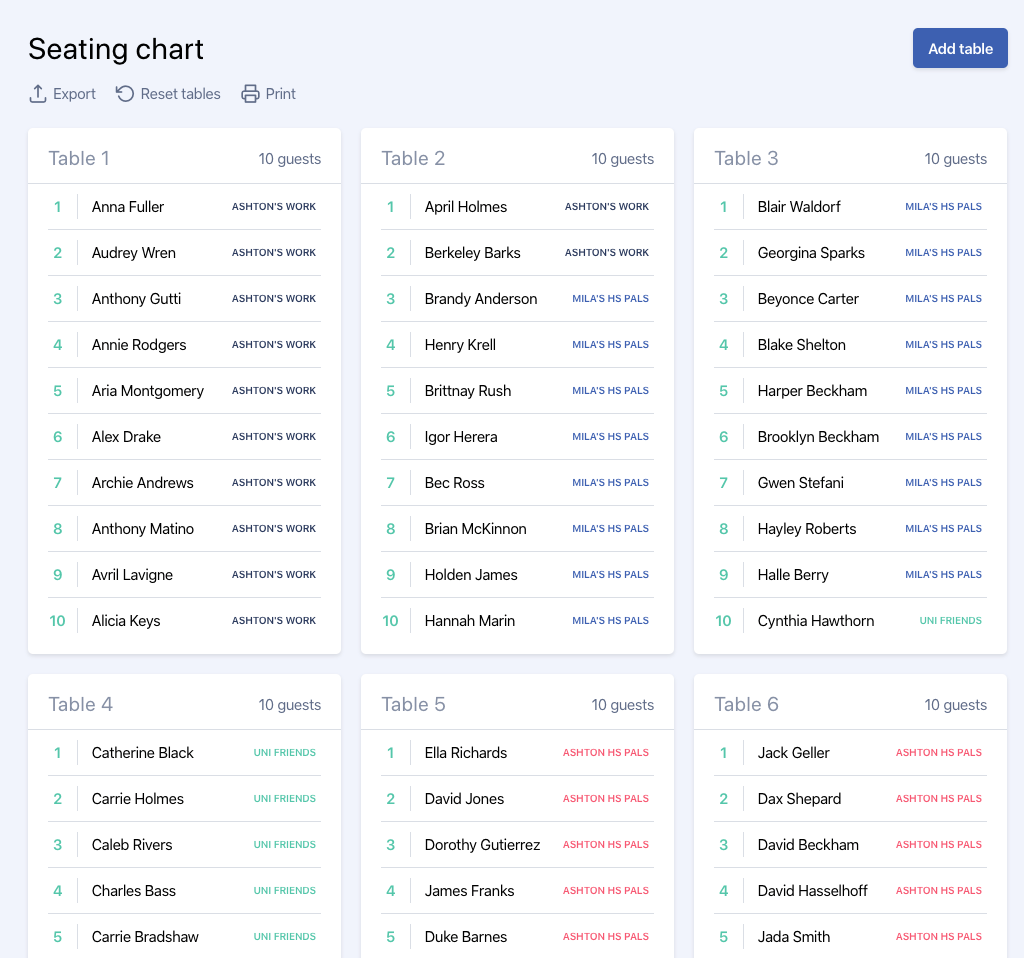The image depicts a detailed seating chart of a city venue. At the top, the seating chart title is prominently displayed. Just below the title, there are options to export, reset tables, and print the chart. Icons representing these functions are positioned to the right of the text. On the left-hand side, there is a section labeled "Our tables," displaying a visual arrangement of tables.

The person has organized six tables, presented in a grid format with three tables in the top row and three in the second row, aligned vertically. Tables 1 through 3 are clearly labeled, each accompanied by a list of 10 names. The names are numbered from 1 to 10 and highlighted in green. These lists are neatly separated by thin vertical and horizontal lines.

Next to each table, there are tabs indicating the groups assigned to them, such as "Ashton's Work" for one table and "Mila's HS Pals" for another. Each tab provides a quick reference to the specific group seated at the table. The remaining tables (4 through 6) also contain lists of guests, but the image cuts off after showing the first five names for each of these tables. The seating chart overall appears organized but not in strict alphabetical order, reflecting a functional and visually clear arrangement for the event.